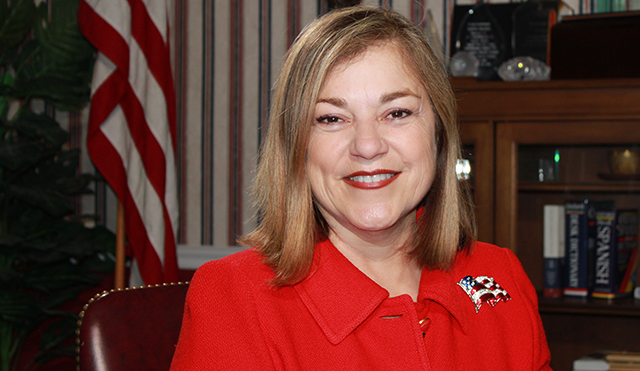In the image, an indoor setting suggests the office of an elected official. At the center of the photograph is a poised woman, potentially in her 50s or 60s, with shoulder-length blonde hair and dark eyes. She is adorned with red lipstick and is wearing a red collared shirt, which prominently features a large American flag pin near its top. She sits comfortably in a dark brown leather chair. The background showcases striped wallpaper along with an American flag on a stand, and to the right, a bookcase with glass doors housing several books, including what appear to be dictionaries, notably a Spanish dictionary. The scene is meticulously arranged, giving a formal and dignified atmosphere.